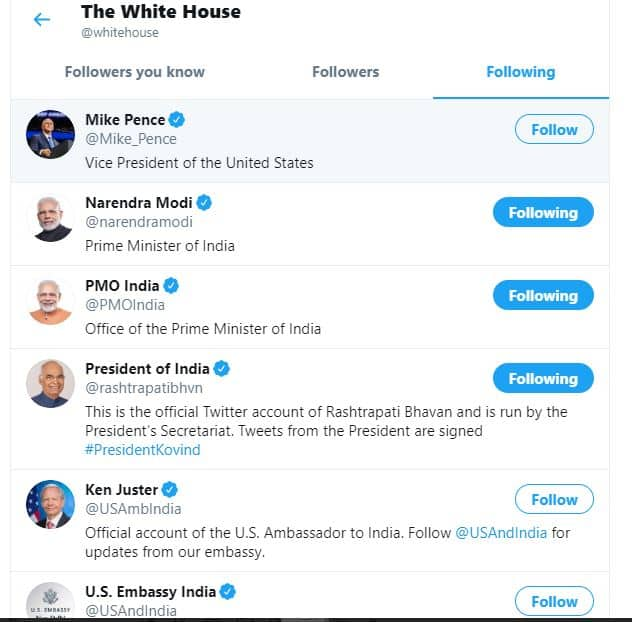The image is a screenshot of a digital interface displaying the official Twitter profile of the White House. At the top of the screen, the header reads "The White House," with the username "@WhiteHouse" displayed directly below it in black print on a white background. To the left of the username, there's a teal arrow icon.

The interface is segmented into three main columns: "Followers," "Following," and a column indicating the action to either follow or unfollow the listed profiles. The "Followers" column is presently empty.

On the left side of the interface, there is a vertical list of circular profile pictures representing various individuals. Each profile is accompanied by details, including the person's name, their Twitter handle, and their professional title, all aligned horizontally.

At the top of the list is Mike Pence, identified with his verified handle "@Mike_Pence" and the title "Vice President of the United States." To the right, there is a button available for users to follow him.

Below Mike Pence is the profile of Narendra Modi, also verified, with the handle "@narendramodi." He is labeled as the "Prime Minister of India," and the interface indicates that this account is currently being followed.

The list continues in this structured format, providing a clear and organized view of notable profiles associated with the White House’s Twitter account.